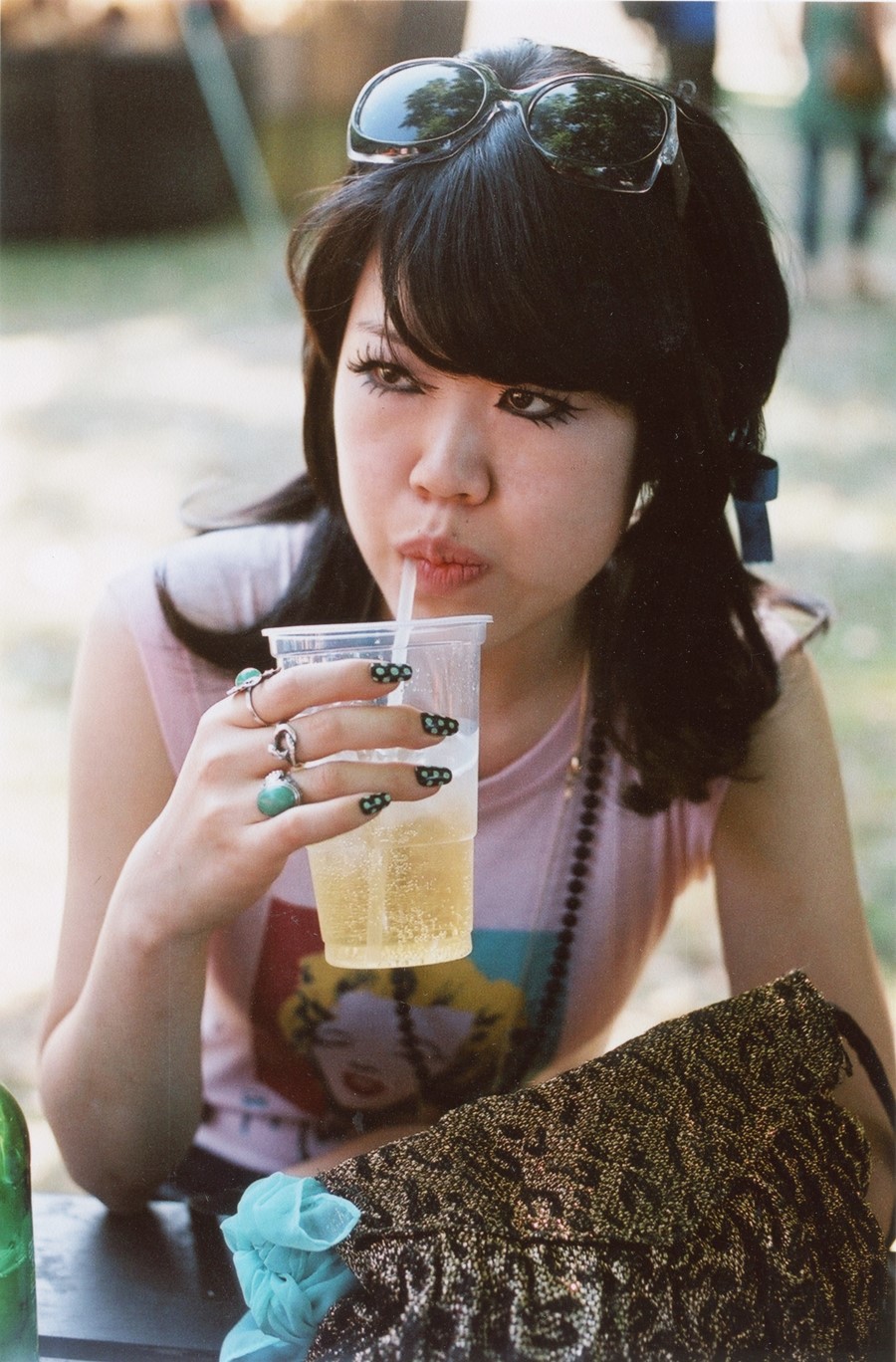In this picture, a young Asian lady with strikingly painted dark eyelashes and pronounced eyeliner gazes intently into the distance. She has dark brown, almost black hair that falls just past her shoulders, styled with bangs. Atop her head rests a pair of reflective plastic sunglasses, capturing a hint of surrounding foliage. She is tastefully adorned with a black beaded necklace and rings on her fingers, with her manicured nails displaying a distinct polka dot blue on black design. 

She is wearing a vibrant pink shirt featuring an image of Marilyn Monroe, accentuated with blown-out colors of red and blue. The woman is sipping a light yellow drink, possibly ginger ale, through a straw from a plastic cup, her lips slightly pursed. There is a bronze and black leopard print purse in front of her, with a turquoise tie dangling from its side. 

With her elbow on a table, she holds the cup in her right hand, featuring three distinct rings: two with turquoise jewels and one silver ring. The background is blurred, suggesting a park setting with a few indiscernible people in the distance, giving the aura of a vintage photograph with muted, pastel tones.